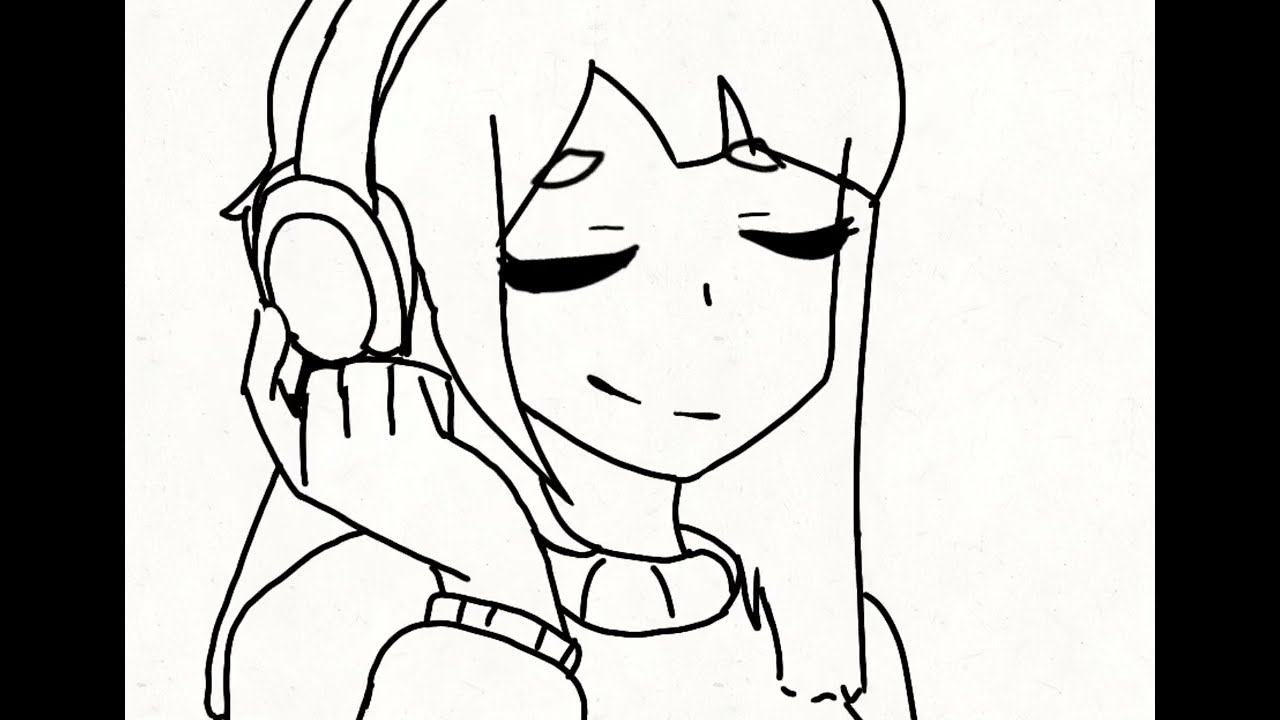This black-and-white cartoon sketch features a young woman or girl wearing over-the-ear headphones, drawn in black pen against a blank white background, framed by thick black borders on the left and right sides. The subject is depicted from just below the shoulders up, with the top of her head cut off by the top edge of the frame. She has straight hair that extends just past her shoulders, with bangs parted in a couple of small sections, and some strands falling in front of her headphones while others flow behind. Her face, turned slightly to the left but mostly facing forward, shows her eyes gently closed with long eyelashes emphasizing a peaceful expression. She sports a slight smile, mainly uplifted on her right side. She wears a long-sleeved sweater, which appears layered over another garment as hinted by the poofy neckline and visible cuffs. Her right arm is raised, with her hand forming a fist except for her extended index finger, which presses against the right earphone, indicating she is absorbed in listening to music.